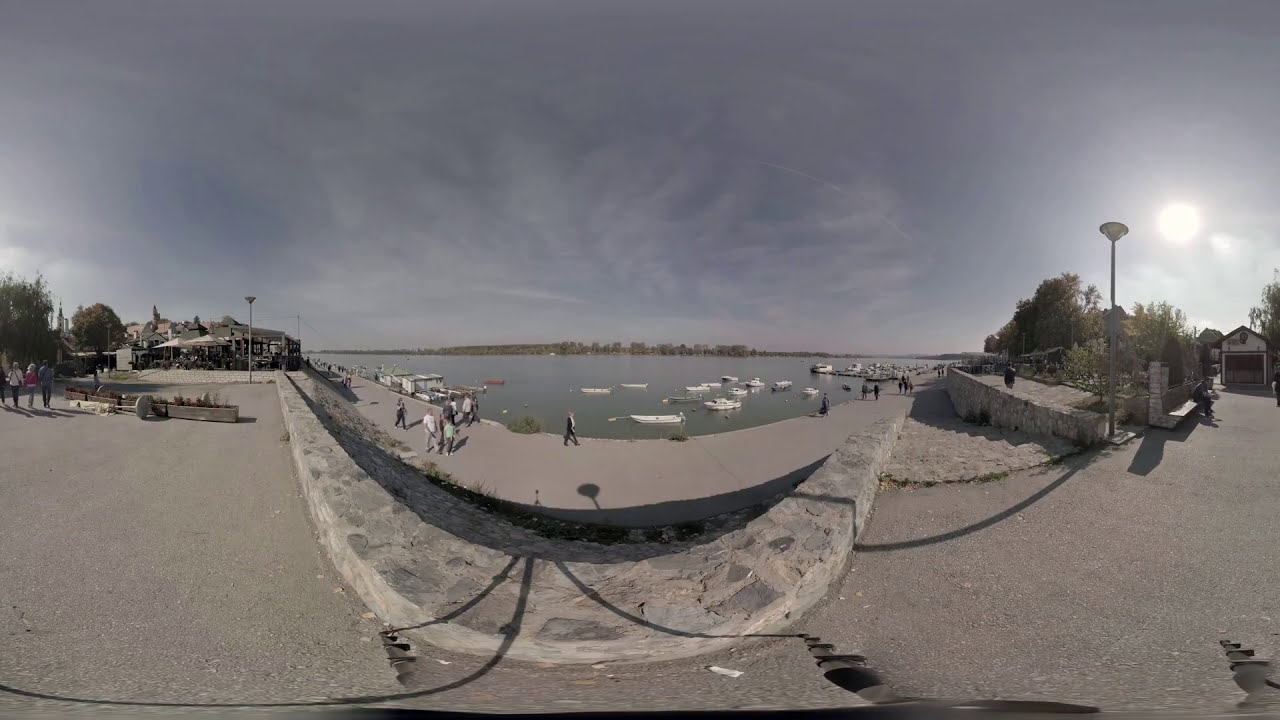This fisheye lens photograph captures a panoramic view of a bustling harbor at dusk, featuring a considerable number of white personal boats floating on a calm, bluish-green body of water. The sky is predominantly gray with some hints of blue, adorned with thin, wispy clouds, and punctuated by a bright white sun in the top right corner, suggestive of an impending sunset or an approaching storm. 

The image is characterized by a gray theme across various elements: the still water, the concrete sidewalks, and the asphalt pathways. These gray pathways curve around the harbor in a U-shape, bordered by a rock wall, alongside which several people are seen strolling. Distant roofs and a scattering of buildings and trees are visible in the background, though they are too far to discern specific details. 

Additional notable features include street lamps positioned on both sides of the photograph, and the entire scene conveys a tranquil yet lively ambiance, typical of a popular tourist spot or gathering space.